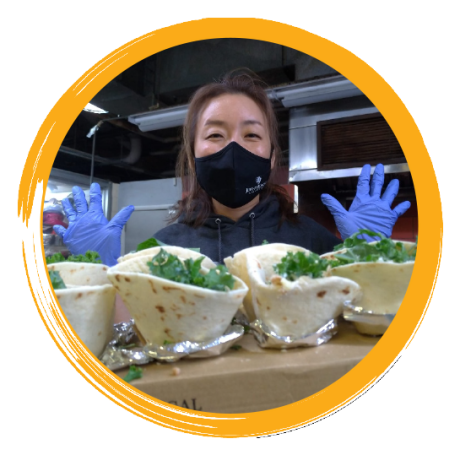In this detailed image, we see an Asian woman with distinctive Oriental features, standing in front of a white background with a large yellow circle framing her from the chest up. She is wearing a black hoodie with the hood down and a black face mask reminiscent of those commonly worn during the COVID-19 pandemic. Her dark brown hair falls below her neck, and she is equipped with blue latex gloves. The woman appears to be in a professional-grade kitchen, as indicated by the presence of a refrigerator and what seems to be a microwave behind her. She is likely preparing food, as in front of her are several items resembling small tortillas or taco shells, each filled with lettuce, possibly chicken, and a white dressing. These filled tortillas are neatly placed on small circles of tinfoil, suggesting that she is meticulously arranging these ingredients. Her arms are raised to head level, perhaps indicating she is in the midst of her culinary task, and though masked, there is a suggestion that she might be smiling.